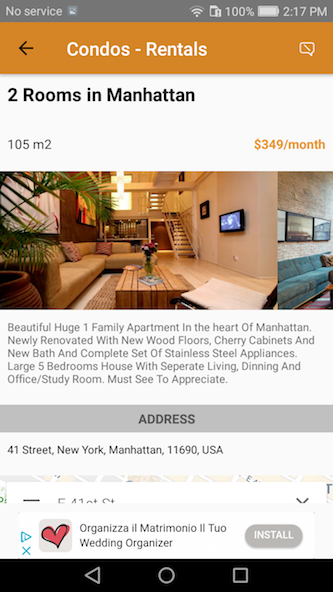Screenshot of an iPhone screen taken at 2:17 PM, displaying no cellular service but a full 100% battery. The image showcases a listing for condo rentals in Manhattan, New York City, specifically on 41st Street. The listing advertises two-room units for the exceptionally low price of $349 per month, which seems unusually inexpensive, suggesting there might be some confusion or a catch regarding the price. Accompanying the listing are images of the condos, which look like luxurious units, featuring amenities such as a swimming pool.